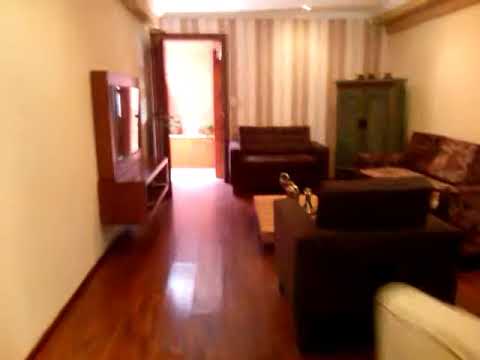This photograph depicts a somewhat out-of-focus interior of a long living room. The room features various pieces of brown furniture, including a pair of dark brown cushioned sofa chairs facing each other and a boxy love seat with a brown floral print. There is a small wooden table with two brass figurines positioned centrally among the seating arrangements. The flooring is a dark reddish-brown hardwood. On the right side of the image, there is a tall, greenish, hutch or cupboard next to the boxy brown love seat, adding a pop of color to the room. On the left side, a tan wall features a brown wooden stand, possibly a TV cabinet. At the far end of the room, an open door reveals a glimpse of another room with white fixtures. Behind the seating area, the wall is adorned with brown and gold striped wallpaper, contributing to the room's warm ambiance. Soft light streams down from an unspecified source, bathing the space in a gentle glow.